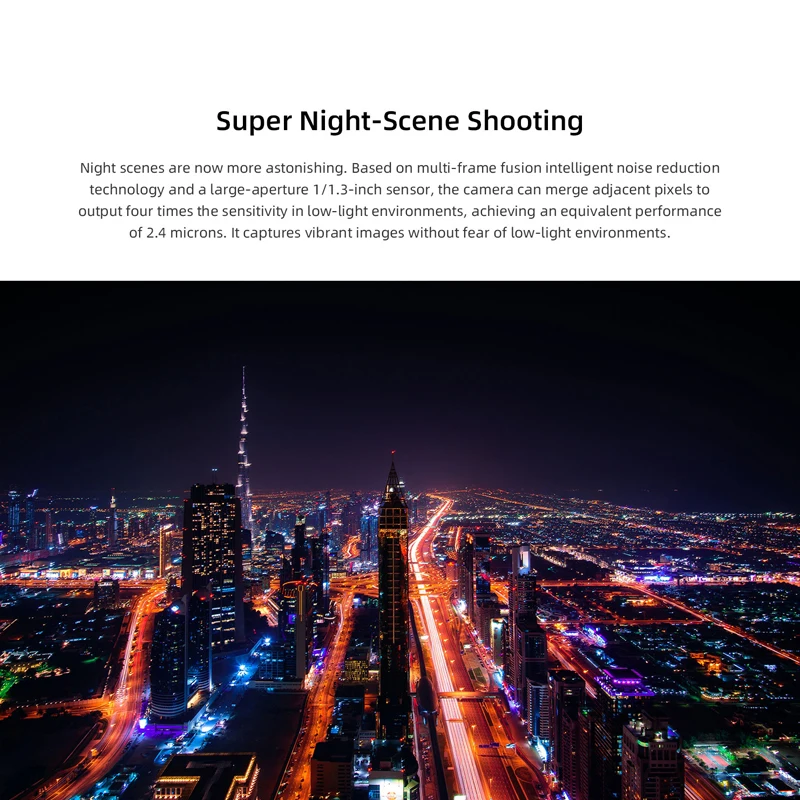The image showcases a captivating, colorful nighttime cityscape with a header overlay in a bold black font that reads, "Super Night Scene Shooting." Beneath it, smaller text elaborates: "Night scenes are now more astonishing. Based on multi-frame fusion intelligent noise reduction technology and a large aperture 1 in 1.3 inch sensor, the camera can merge adjacent pixels to output 4 times the sensitivity in low-light environments, achieving an equivalent performance of 2.4 microns. It captures vibrant images without fear of low light environments."

The bustling downtown area extends far into the distance, hinting at a sprawling metropolis possibly similar to Hong Kong, but not identifiable as New York due to the mix of moderately tall and very tall buildings. The streets are illuminated in a golden hue, likely from streetlights, rendering a busy atmosphere with visible car movement. The city lights vary in color, contributing to a vivid, lively scene. Amidst the dark sky, there's a subtle red and bluish-violet glow near the horizon, possibly from the city lights. Prominently, a towering, pointed building stands in the background, while in the foreground, at least four skyscrapers with lit windows dominate the view, surrounded by shorter buildings, all contributing to a stunning and dynamic nightscape.